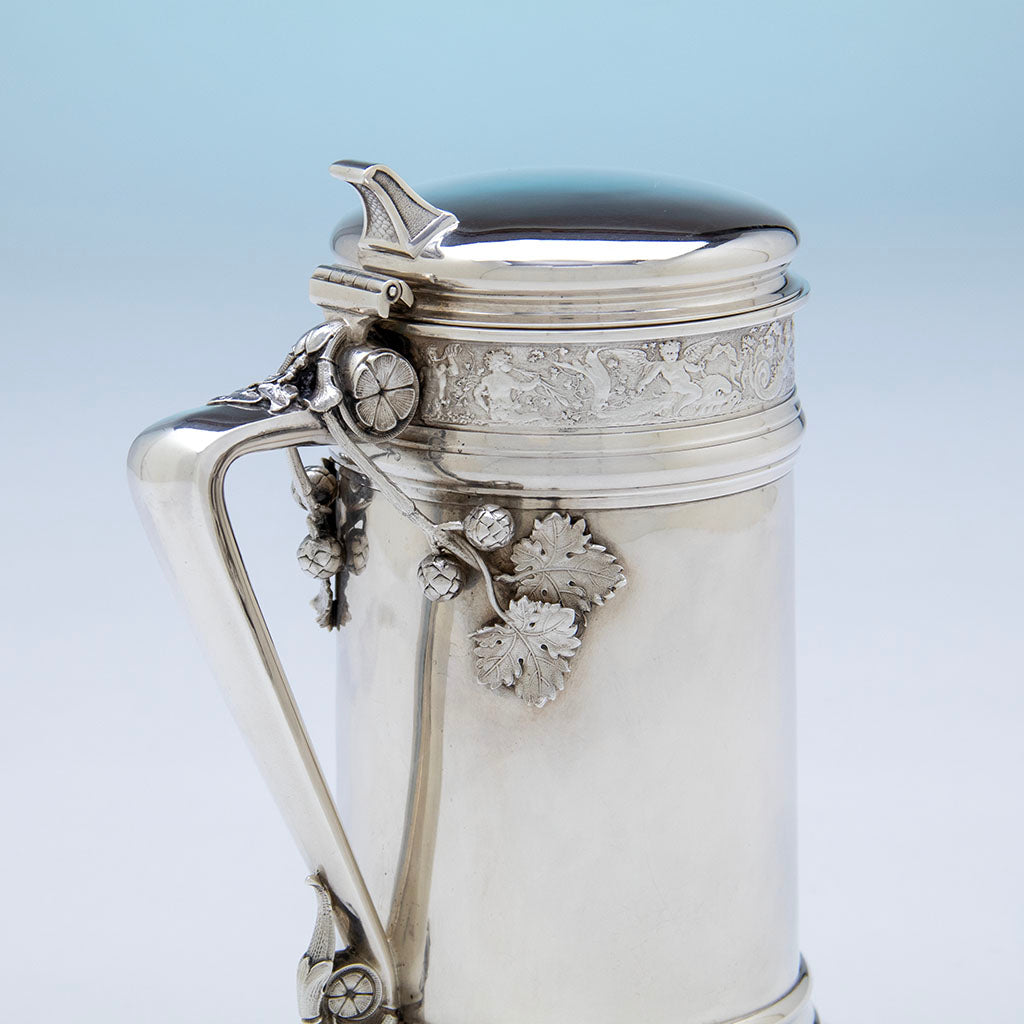The photograph showcases a highly detailed, polished silver antique beer stein, likely from the late 1800s to early 1900s. Set against a gradient background that transitions from pale blue at the top to white at the bottom, the stein is presented at an angle highlighting its intricate craftsmanship. The straight handle, featuring a curvature towards the mouth of the stein, is adorned with ornate designs of silver oak leaves and small oak balls. The top of the handle includes a functional thumb clasp, allowing the lid to be easily lifted. Around the lip of the stein, an elaborate one-inch-wide silver mural depicts carved figures that appear to be cherubs or angels, adding to its exquisite detail. The lid itself is polished to such a degree that it reflects its surroundings.